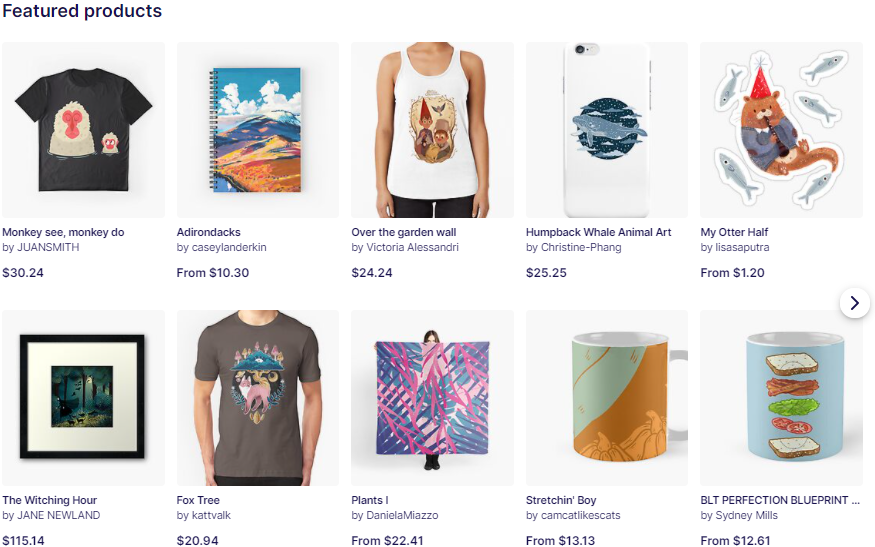The image depicts a computer screen showcasing products available for sale, arranged in two rows of five products each. Each product is displayed within a light gray square, featuring a color photo of the item, alongside its description, the artist's name, and the price. The overall background of the screen is white, with the phrase "Featured Products" written in dark letters at the top left.

### Top Row (Left to Right):
1. **"Monkey See, Monkey Do" by Juan Smith** - This item is a dark shirt adorned with pictures of monkeys, priced at $30.24.
2. **"Adirondacks" by Casey Landerkin** - A spiral-bound notebook with a picturesque cover featuring clouds and an outdoor scene, starting at $10.30.
3. **"Over the Garden Wall" by Victoria Alessandri** - A sleeveless white tee displaying images of gnomes, available for $24.24.
4. **"Humpback Whale Animal Art" by Christine Fang** - A white cell phone case showcasing a picture of a whale on the back, priced at $25.25.
5. **"My Otter Half" by Lisa Sputra** - An artwork featuring an otter wearing a red hat with little fish around it, starting at $1.20.

### Bottom Row (Left to Right):
1. **"The Witching Hour" by Jane Newland** - A framed portrait with a black frame and white mat, depicting a dark woods scene, priced at $115.14.
2. **"Fox Tree" by Kat Valk** - A gray shirt featuring a large picture of a fox, available for $20.94.
3. **"Plants One" by Daniela Meazzo** - A woman is shown holding a large square cloth adorned with blue and pink leaves against a light pink background, starting at $22.41.
4. **"Stretchin' Boy" by Camcat Like Scats** - A drinking mug decorated with pumpkins and aqua tones, priced at $13.13.
5. **"BLT Perfection Blueprint" by Sydney Mills** - A light-blue mug illustrating the ingredients of a BLT sandwich, available for $12.61.